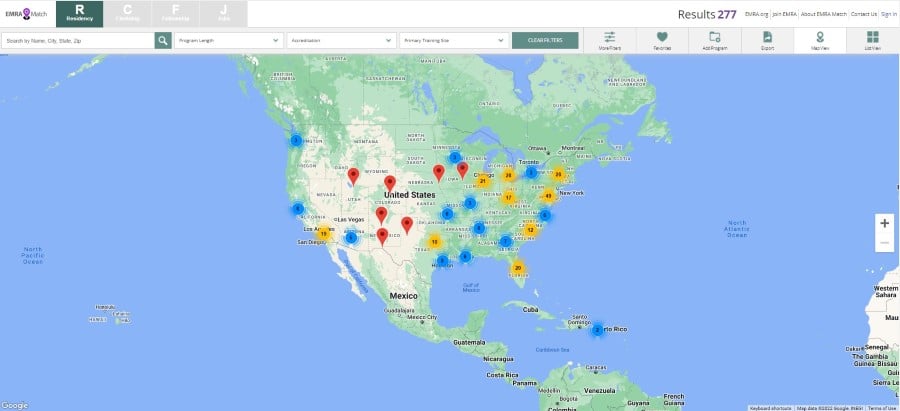The image displays a detailed map encompassing the entire United States along with significant portions of Canada and Mexico, and the upper reaches of South America, specifically highlighting Venezuela, which is labeled in the largest and clearest text. Scattered across the map are various navigation markers typically found on GPS systems, primarily red in color. These markers are concentrated in the central region of the U.S., with additional clusters in the southern states and a prominent grouping along the East Coast. There are also several circles in blue and yellow, each containing specific numbers, adding a layer of information to the map's visual data. The text on the map is somewhat blurred, making it challenging to decipher specific details other than the notably clear "Venezuela."